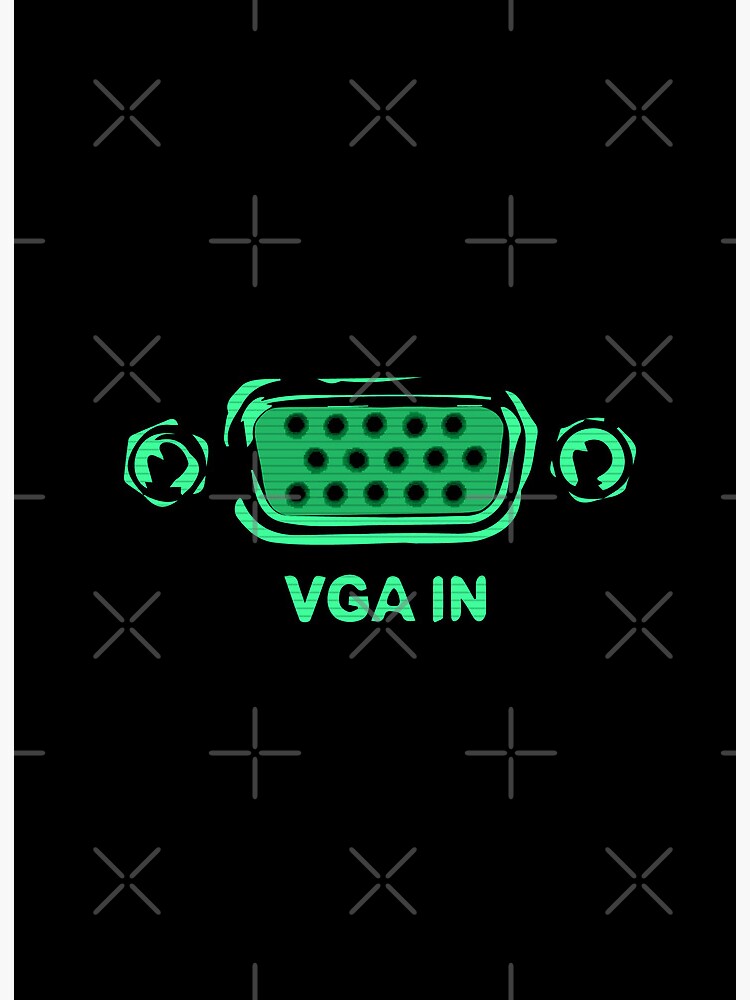The detailed artistic image features a meticulously hand-drawn illustration of a VGA port, rendered in vibrant neon green ink. The port prominently centers in the image, showcasing its characteristic trapezoidal shape with an array of multiple small pinholes. Flanking each side of the pinholes are two larger holes designed for screws, meant to securely fasten a VGA cable to a monitor or device. Below the graphic representation of the VGA port, the letters "VGA-IN" are inscribed in bold, neon green bubble letters. The entire composition stands against a stark black background adorned with a vertical pattern of light gray X's and crosses, adding a rhythmic texture to the backdrop. This visually striking piece captures the essence of retro technology with a modern, artistic twist.